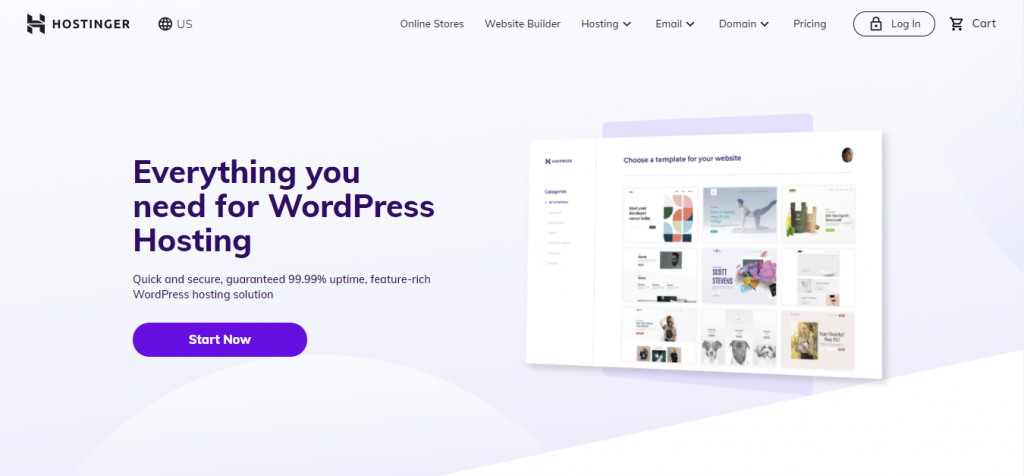Set against a white and lavender background, this screenshot features the upper left corner of a website interface. In the forefront, there is a "H" logo, followed by the black text "Hostinger." To the right, a circular icon displays the word "US." Spanning the top of the interface, the navigation menu includes options labeled "Online Stores," "Website Builder," "Hosting" (with a pull-down menu), "Email" (with a pull-down menu), "Domain" (with a pull-down menu), "Pricing," a "Login" action button, and a shopping cart icon.

Centered prominently below the navigation bar is the bold text stating, "Everything you need for WordPress hosting." Underneath, in smaller text, it reads, "Quick and secure, guaranteed 99.99% uptime, feature-rich WordPress hosting solution." Below this description, a dark purple action button is displayed, featuring white text that invites users to "Start Now."